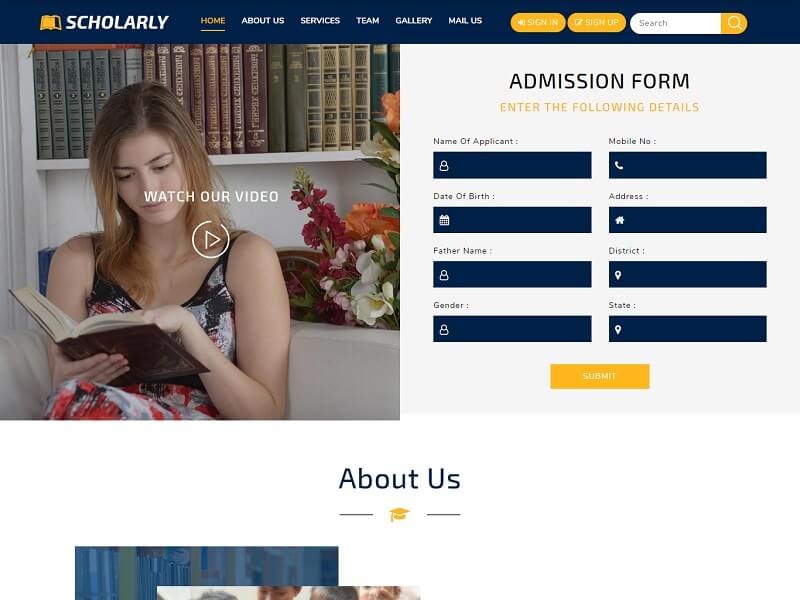**Website Description: Scholarly Home**

The image falls under the category of websites and represents a section from a page titled “Scholarly Home.” At the top of the page, there's a dark blue navigation bar. In the left-hand corner of this bar, there is a yellow book icon alongside the word "Scholarly" in white letters and the word "Home" in yellow letters, which is underlined. The bar also features a navigation menu with the following options in white text: About Us, Services, Team, Gallery, Mail Us. On the right-hand side of the bar, there are two yellow buttons labeled "Sign In" and "Sign Up," alongside a search bar.

Below the navigation bar, on the left-hand side, is an inviting picture of a young lady sitting amidst bookshelves and flowers, engrossed in reading a book. She is wearing a dress, enhancing the serene and studious environment. Centrally placed on her image is a play button with the text "Watch Our Video." To the right of this picture, there is a form labeled "Admission Form." The form prompts the user to enter the following details: Name of Applicant, Mobile Number, Date of Birth, Address, Father's Name, District, Gender, and State. A "Submit" button is located at the end of the form.

Beneath this, there is a section titled "About Us," initiating the further content of the page.